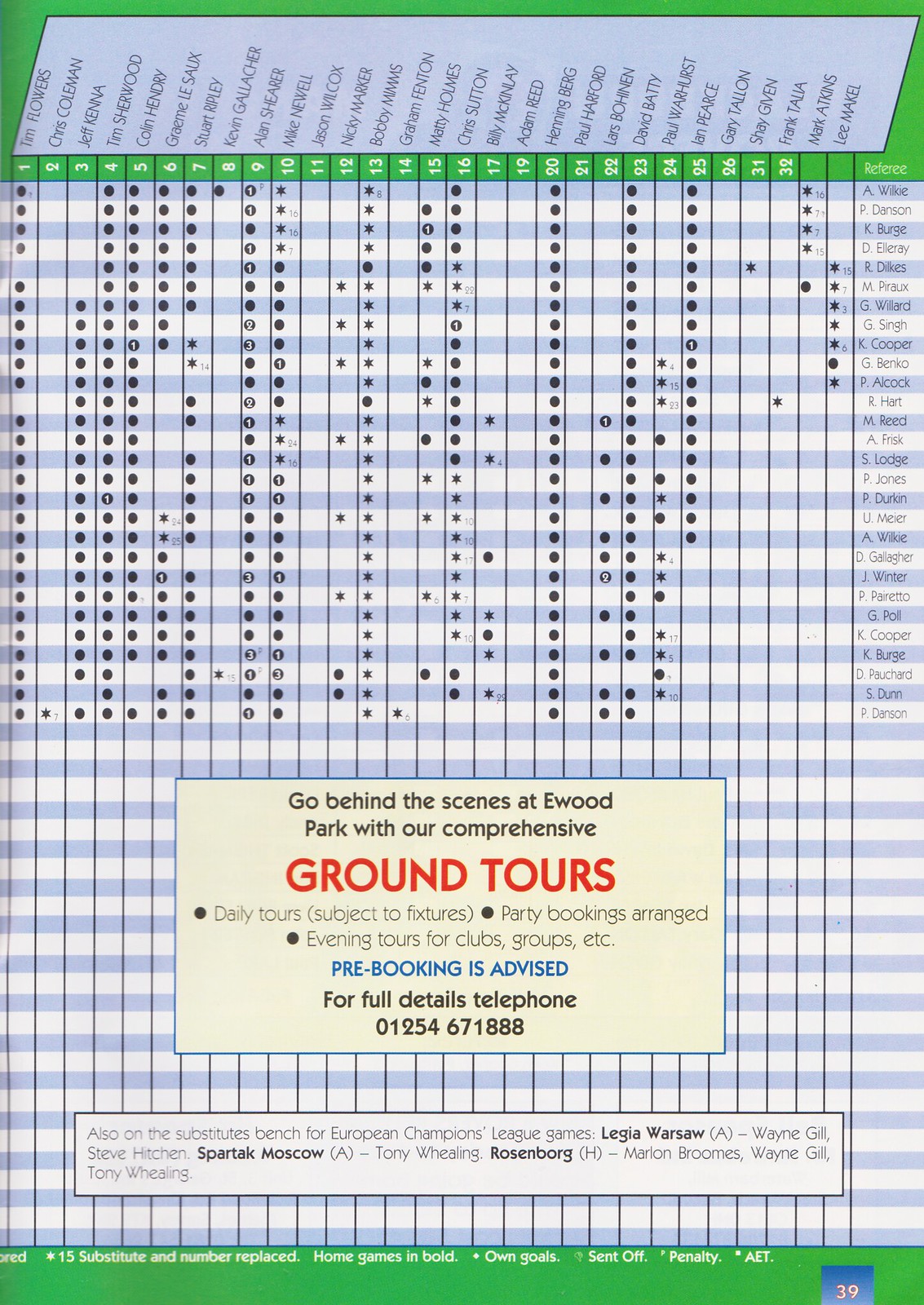The image is a promotional chart for comprehensive ground tours at Ewood Park. The top part of the document, approximately an inch and a quarter tall, features a band with names of various stops against a green background. Below this band, the main body consists of a detailed blue and white chart connecting rows of stop names with columns of times or other attributes, indicated by black dots in the corresponding boxes. The bottom third of the chart is notably sparse, with the absence of dots indicating no stops.

Dominating the lower middle section is a central box measuring about 2 inches tall by 4 inches wide, containing the main promotional message in red and pale black lettering. The message reads: "Go behind the scenes at Ewood Park with our comprehensive Ground Tours," with 'Ground Tours' in capital red letters. Bullet points detail daily tours subject to availability, party bookings, and evening tours for clubs and groups, ending with a note in pale black stating "Pre-booking is advised" and a contact telephone number. 

Near the bottom of the image is another rectangular green box, about 1.5 inches tall by 6 inches wide, containing miscellaneous terms such as 'European Champions League,' 'substitute,' 'home games,' and 'own goals,' though much of this text is not fully legible. This entire document seems to be designed as a handout or flyer, approximately 5 inches wide and 8 inches long, to inform visitors about the scheduling and details of the Ewood Park ground tours.